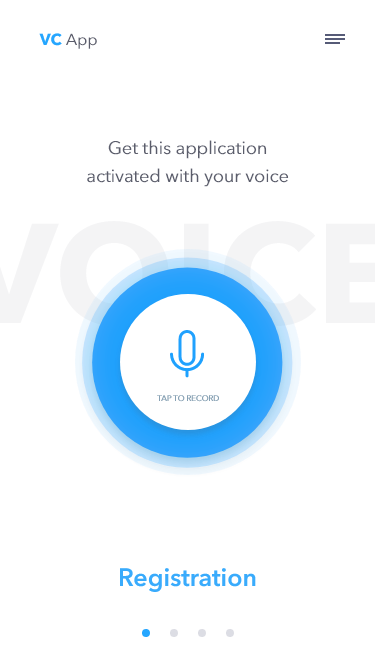This image showcases a user interface for a voice control application. At the top left corner, the text "VC app" is prominently displayed, with "VC" highlighted in blue and "app" in gray. To the right of this text, there are three horizontal black bars; the top two bars are longer, while the bottom bar is shorter, likely representing a menu icon.

Beneath the title, centered on the screen, is the text "Get this application activated with your voice," emphasizing the use of voice commands. The word "voice" spans the full width of the highlighted text and appears in a gray, slightly faded font.

In the middle of the image, there is a prominent blue circle containing a smaller white circle with a blue microphone icon inside. The microphone symbol resembles an upright pill with a smiley face underneath and a small stem in the center, symbolizing the mic stand. Below this icon, the phrase "Tap to record" is displayed, indicating the interactive feature of the app.

At the bottom of the screen, in blue and centrally aligned, is the word "Registration." Below this text are four dots arranged in a horizontal line. The leftmost dot is blue, indicating the current step in the process, while the three subsequent dots are gray, suggesting incomplete steps.

Overall, this is a detailed user interface for a voice command application or a request to enable microphone functionality within an app or website.